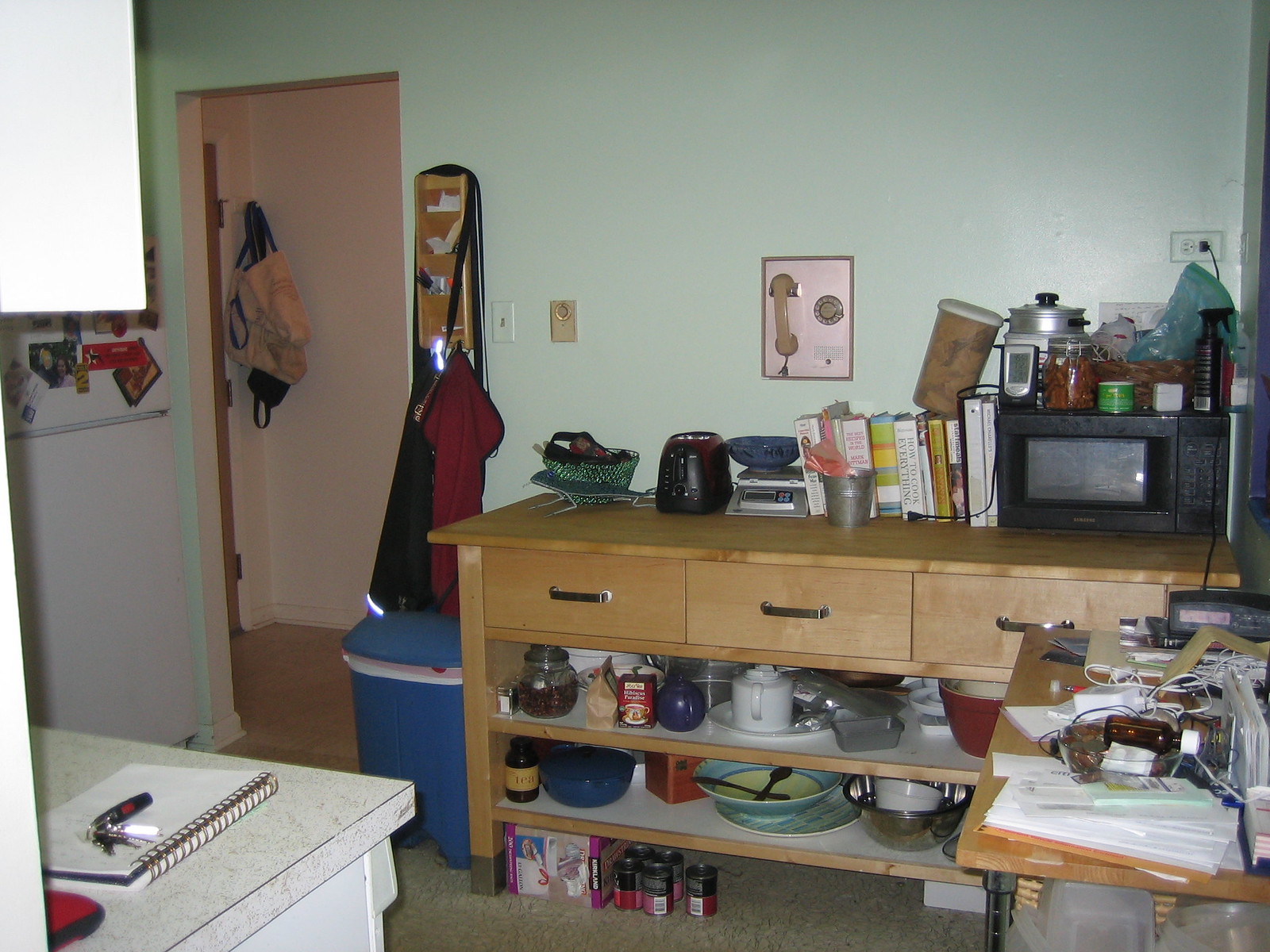The image captures a detailed kitchen scene with various objects and colors. The flooring is a greenish hue, setting the base for the room. A brown shelving unit with silver-metal drawers holds two shelves where black and purple jars sit beneath it, next to a box. Through a doorway in a light green wall, there is a white door with black handles and a whitish bag hanging on it.

To the far left, a white refrigerator is adorned with reddish and bluish magnets. A white speckled countertop occupies the bottom left corner, on which a white book with red connectors lies beside a pair of keys; one keychain is black with a red spot, likely car keys. Near the doorway, a blue garbage bin is visible, and a black and red top hangs from a brown envelope holder.

A light fixture is mounted next to the light switch, and a nearby temperature gauge switch is light brown. Moving to the right, a light brown phone sits on a square metal plate with a rotary dial beside it. Adjacent to this is a square brown object resting on top of a stack of books. Further right, some jars are positioned on top of a black microwave with a clear screen.

The right side of the room features a brown table with black legs, cluttered with white papers and some mixed white papers, alongside plates and bowls in the shelving beneath. On the bottom shelf, a silver bowl stands out next to a blue and yellow bowl with black spoons inside, a red box, a blue bowl, and a black bottle with a yellow stripe. Above, a white kettle for tea is also visible, completing the scene.